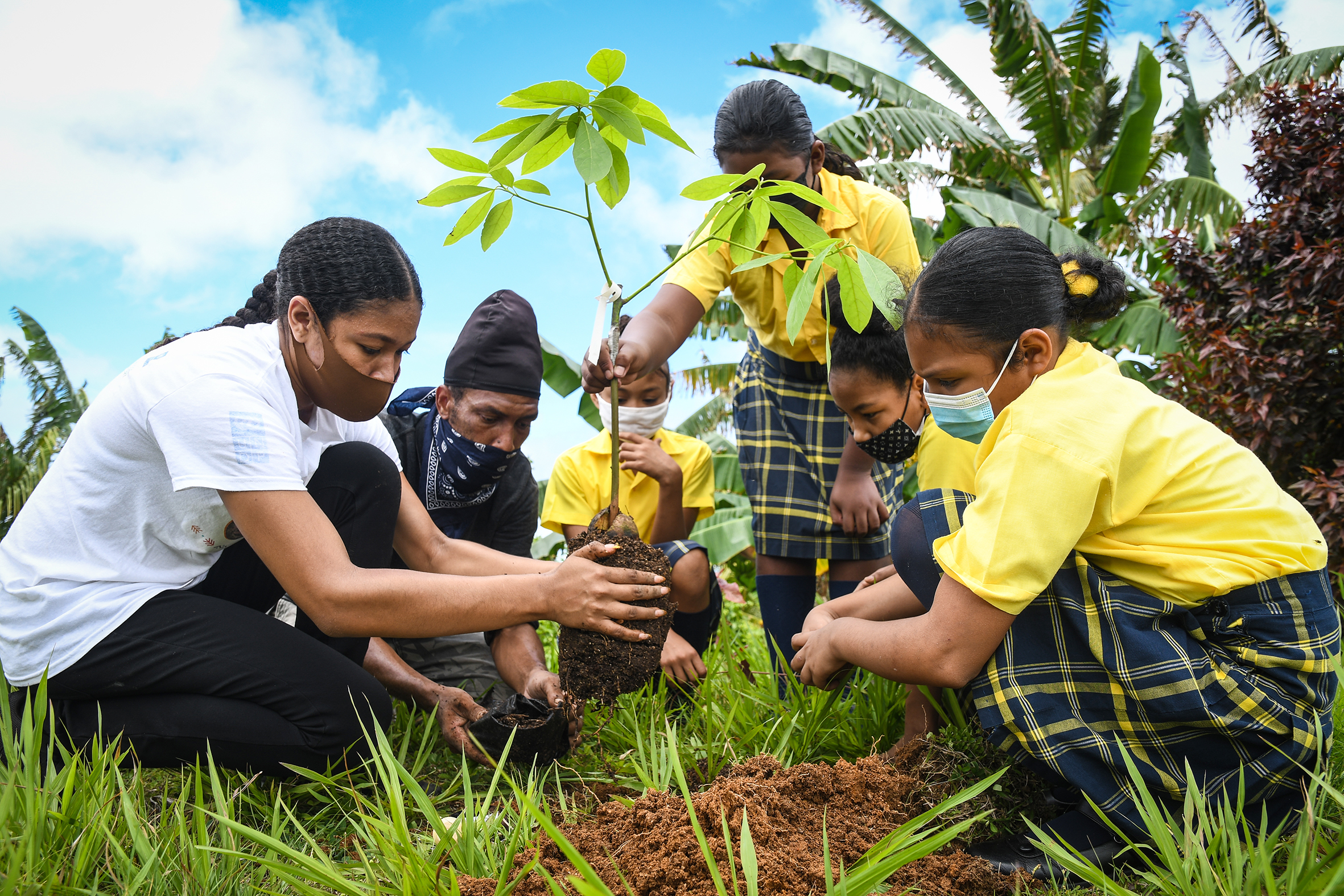This colored photograph captures six people, mostly young women and children, engaged in planting a seedling outdoors. The group, likely from Southeast Asia, includes one man, second from the left, wearing a blue shirt, a soft beanie hat, and a bandana mask. He appears to be placing fertilizer into a hole in the ground. Surrounding him are five young individuals, all wearing yellow shirts and blue and yellow plaid skirts, except for one woman in a white shirt and black pants. 

The children, central to the image, are assisting with the planting: one girl holds the plant's dirt ball over a mound of soil, while another girl's hand grips the stem, distinguished by a white ribbon tied to it. They all wear various types of masks, emphasizing the COVID-era setting. The background features palm trees, clear skies with a few clouds, and uncut grass along with some ferns, adding to the lush, natural scenery of the planting site.